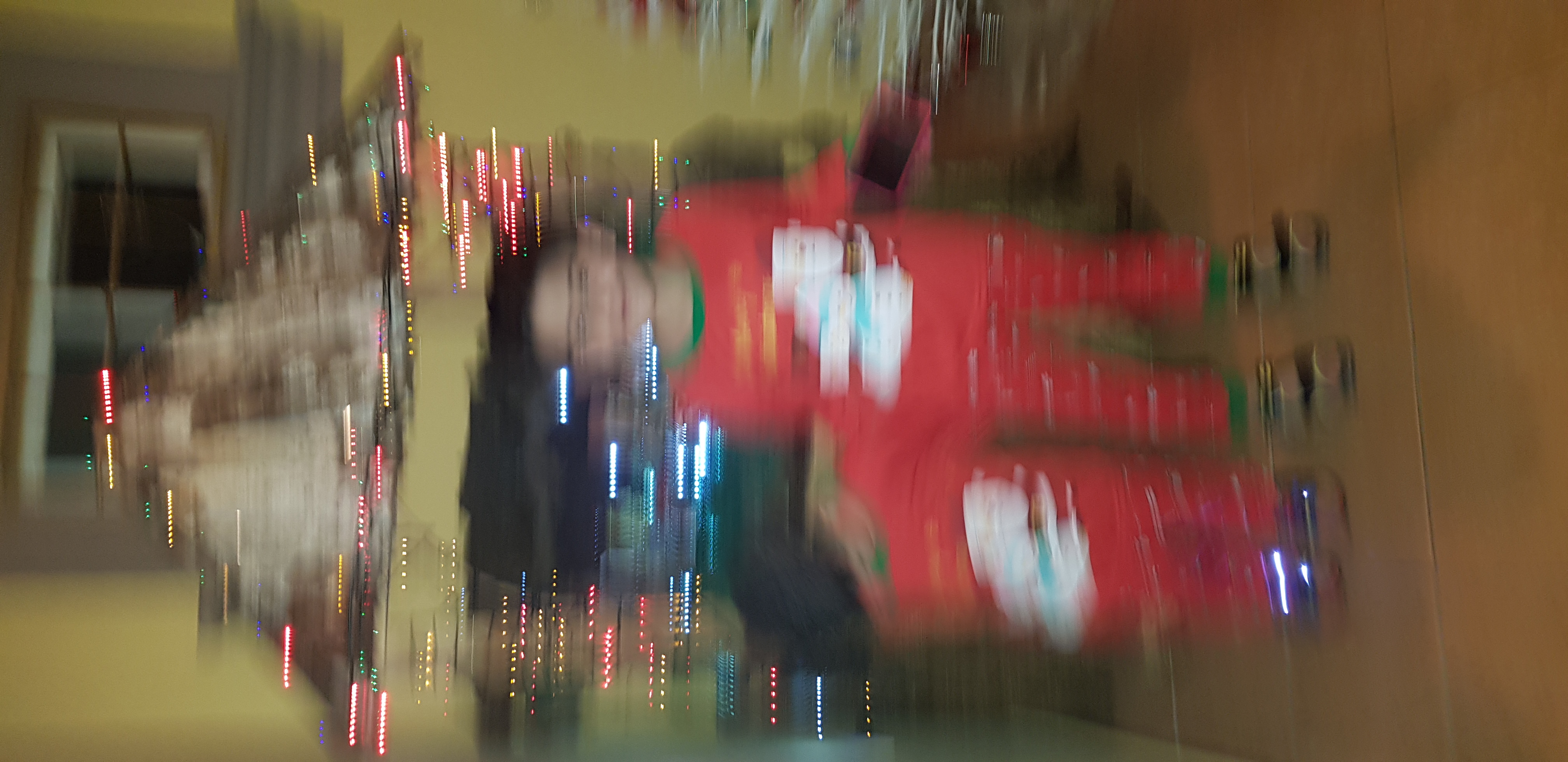Two little boys stand in front of a display of Christmas lights in a photograph that is noticeably blurry and rotated to the left. The boys are dressed in matching red Christmas pajamas, each adorned with a Santa Claus graphic, and are wearing sandals on their feet. Both children have short brown hair. The background features glowing Christmas lights arranged in what appears to be a triangular, pyramid-like shape. The walls behind them are painted yellow, and there is a rectangular mirror visible on the very left side of the image.